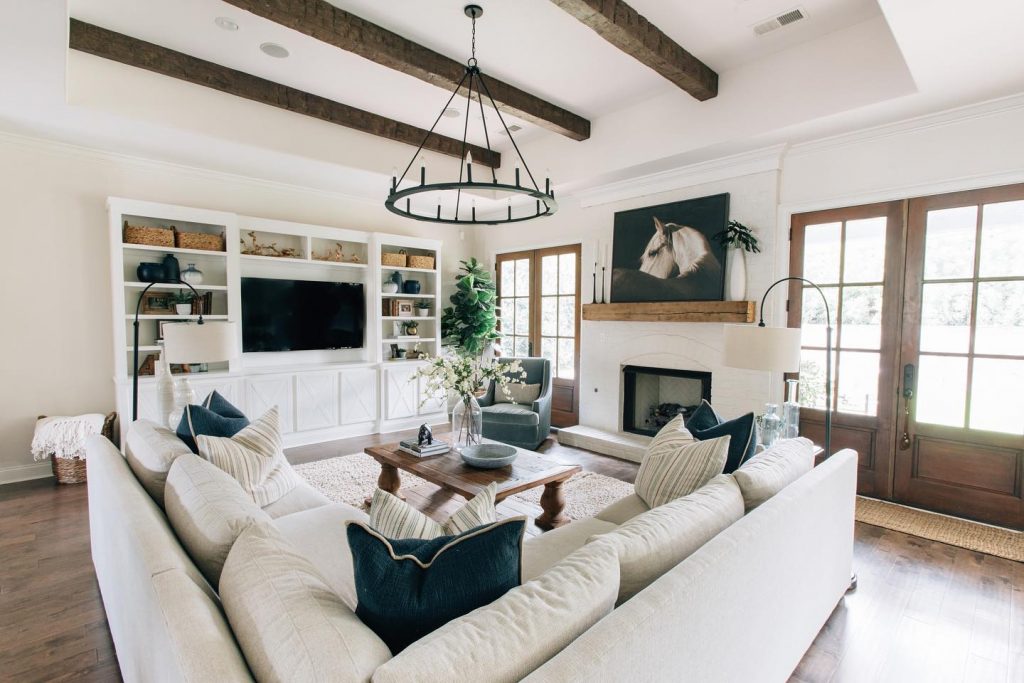This image showcases a luxurious, well-appointed living room with a harmonious blend of comfort and elegance. The room features a polished medium-color hardwood floor that complements the white painted walls and ceiling, which is adorned with wooden beams. A black, wagon wheel-like chandelier with candle-style lights hangs centrally, highlighting the sophisticated ambiance.

On one wall, there are two large doors framed by wood and equipped with glass panes, allowing ample daylight to flood the room. Between these doors is a white fireplace with a wooden mantel, crowned by a striking black and white photograph of a horse. The mantel is flanked by large candles and small white flower vases, enhancing the decorative charm.

To the left of the fireplace, there are built-in white cabinets and shelves filled with books, flower vases, and various artifacts. Directly ahead, a large flat-screen TV is mounted on the wall, above additional closed white cabinets that provide clean and practical storage.

In the center of the living room sits an L-shaped sectional sofa upholstered in white, punctuated with an array of cushions in black, white, and blue, along with striped patterns featuring light gray and light brown accents. A white rug lies beneath a brown wooden coffee table that holds a gray bowl, magazines, and a flower vase with a large, indoor plant standing nearby.

Additional details include a gray single sofa near one of the doors and a substantial lamp placed alongside the sofa set. A subtle basket with a white cover adds a touch of homely warmth, completing the detailed and inviting decor of this premium living space.